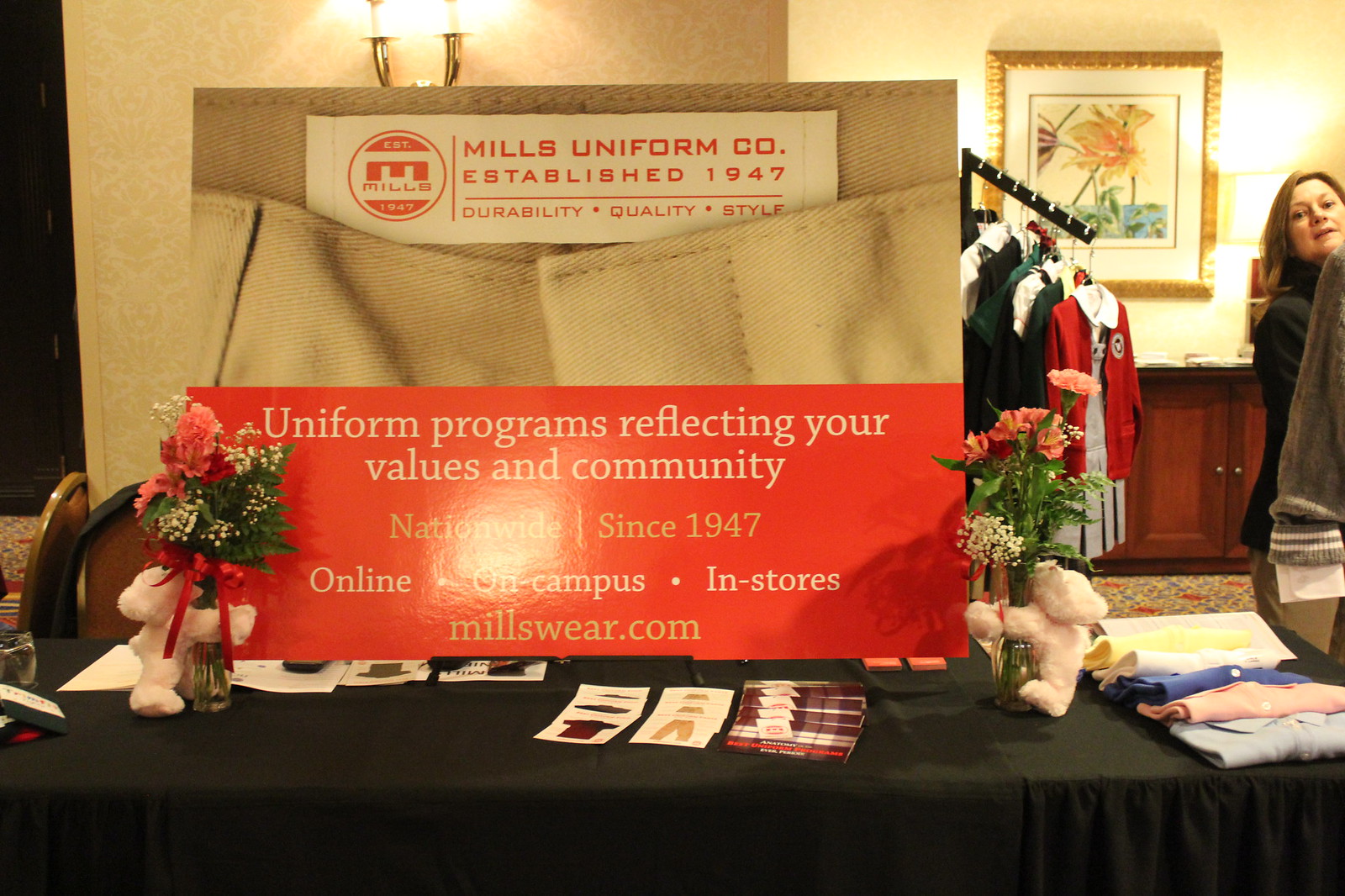This indoor photograph captures an informational display table set up by the Mills Uniform Company at a convention. The table, draped with a dark brown-green tablecloth, features several lines of pamphlets spread out along its front edge. Behind the pamphlets stands a prominent red sign that reads, "Uniform Programs Reflecting Your Values and Community, nationwide since 1947, online, on campus, in stores, Millsware.com." Flanking this sign are two vases with flowers and attached stuffed bears. On the right end of the table, there are several pieces of folded clothing arranged in a row.

Above the display is a white banner with red print stating, "Mills Uniform Company, established 1947, durability, quality, and style." The Mills Uniform Company’s symbol—a red circle with an 'M' and the word 'Mills' underneath it—is also visible. Behind the table, a nearby wall on the left has a hanging light, while the right-hand side of the photograph shows a room with a woman interacting with clothing on display racks. The racks feature various pieces of clothing, including a red jersey and other items in blue and white, highlighting the company's product range. A framed picture of a flower is seen in the background, adding to the decor of the setting.